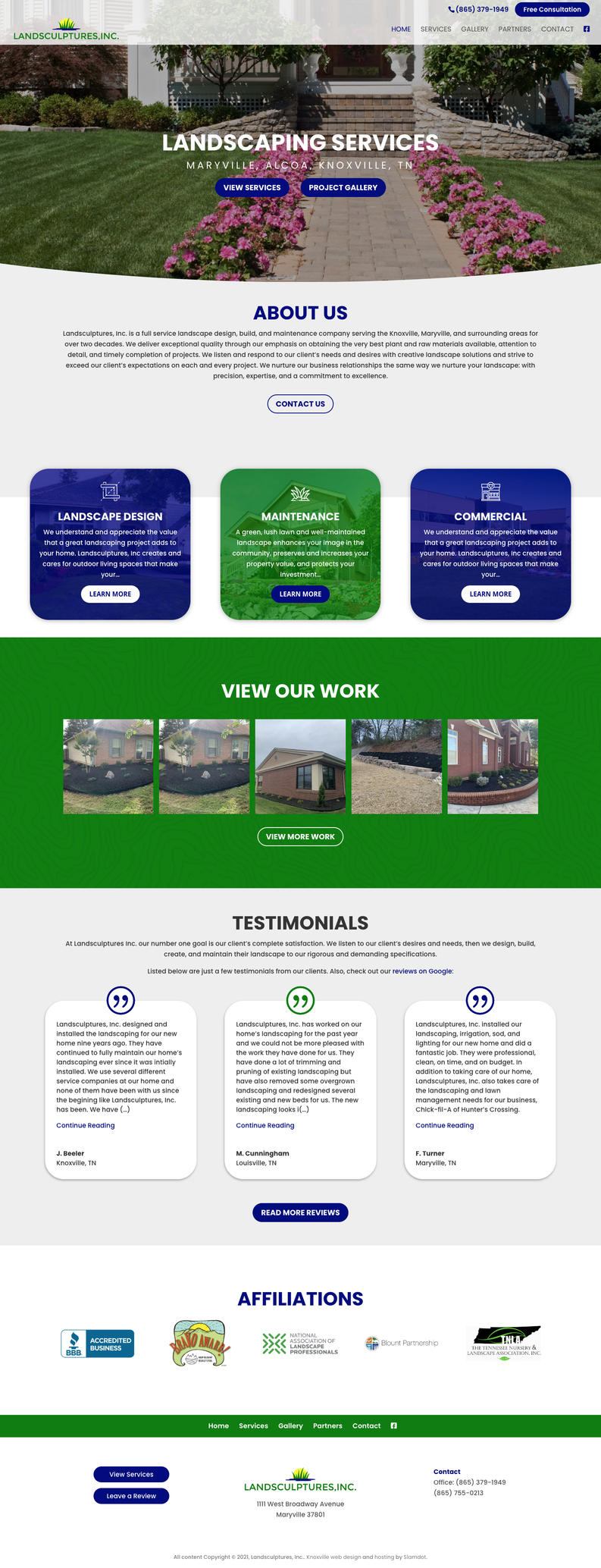This detailed landing page for a landscaping services company prominently features a top section with a visually appealing image showcasing their landscaping work. Immediately below this image is a brief "About Us" section. The page is segmented into three distinct, labeled boxes. The first box, highlighted in blue, details their "Landscape Design" offerings with white text. The second box, also in blue, focuses on "Maintenance" for both residential and commercial properties. The third box, a green square, invites visitors to "View Our Work," linking to a gallery of their projects. Further down, the page features a section for testimonials with three displayed initially, but users can click to read more. Affiliation logos of trusted organizations, such as the Better Business Bureau (BBB), are showcased, enhancing the company's credibility. The bottom of the page is anchored by a green bar. Overall, the design highlights trust and professionalism, making it easy for visitors to find relevant services and client feedback.